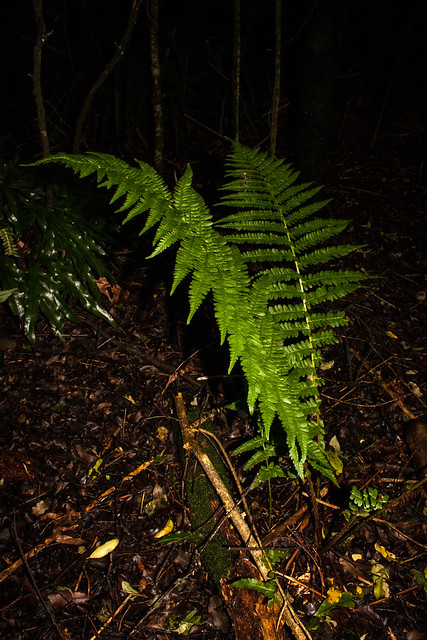This detailed nighttime photograph captures a lush forest floor after a rainstorm, featuring two prominent fern leaves as the central focus. The vibrant green ferns, glistening with moisture, stand out sharply against the darker, less colorful background, likely due to the use of flash photography. Surrounding the ferns, the ground is muddy and damp, littered with saturated sticks and forest debris. Additional plants, including a shiny, wet leaf to the back left, add depth to the scene. The background is a shadowy mix of indistinct trees or weeds, barely visible in the dim light. The overall color palette includes various shades of green and brown, punctuated by occasional hints of yellow and white highlights from the wet foliage.